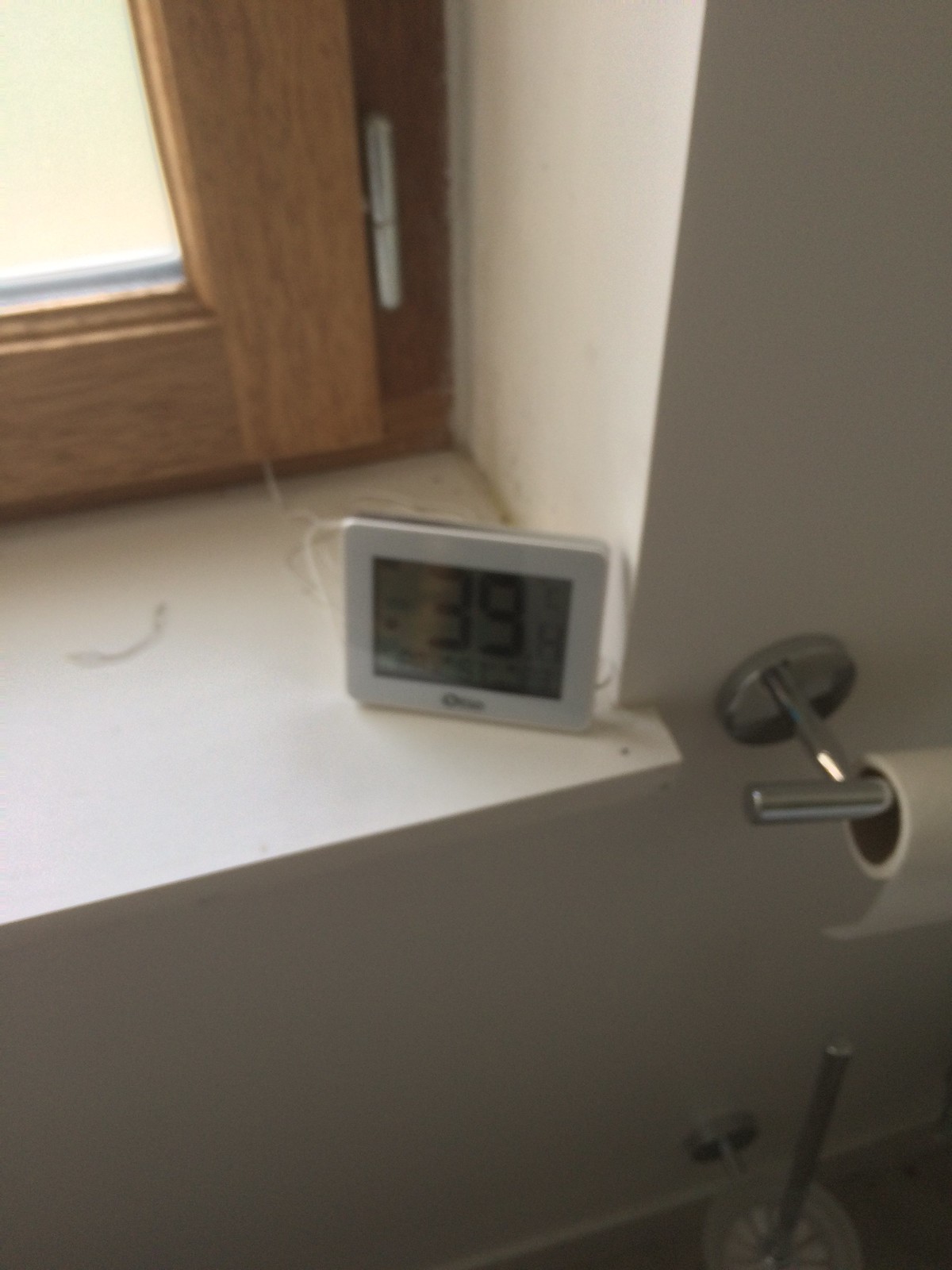The image, though blurry, captures an intimate view of a restroom. At its center is a machine with a digital screen displaying the number 39. This machine is positioned on a shelf attached to a wall. The wall, painted white, serves as a subdued backdrop. To the right side of the image, slightly below the machine, a metallic toilet paper holder is fixed, with a roll of toilet paper resting on it. Directly beneath the holder, a metal toilet brush wand stands in its holder. In the background, there appears to be a wooden-framed window connected to a hinge, adding a rustic touch to the otherwise utilitarian space. The wall continues in its white simplicity, and though a small portion of the floor is visible, its exact color remains indiscernible, presenting itself as a muted, neutral shade.